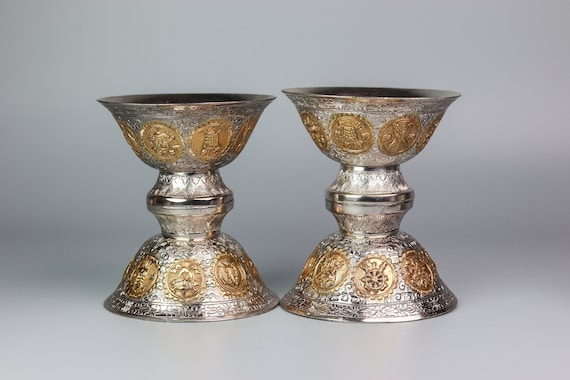The photograph showcases four ancient, ornate bowls, resembling goblets, displayed on a stark white table with a white background. Arranged in a unique mirrored fashion, two bowls are placed upside down with the other two stacked on top, creating a symmetrical and reflective composition. Each bowl, primarily silver with some tarnish, features an hourglass shape—narrow in the middle and wider at the top and bottom. Encircling the bowls are intricate gold accents, including circle-shaped designs that resemble small coins or pennies, adorned with detailed floral and image motifs. The bowls have a round foot base, and towards the black, hollow interiors, the silver surface transitions into the decorative golden patterns that add to the overall historical allure of the artifacts.